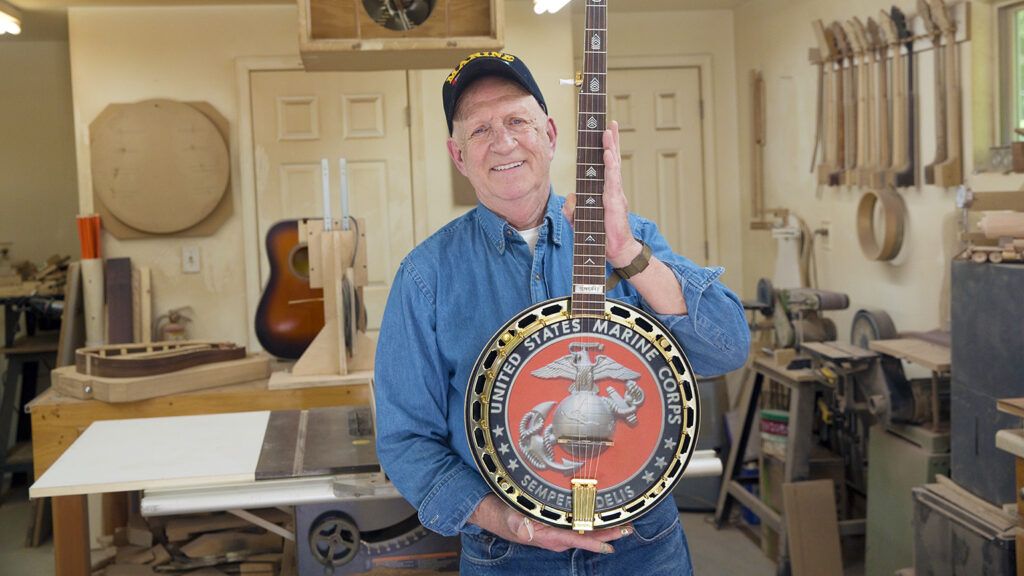In the image, an older Caucasian man is proudly showcasing a handcrafted banjo in what appears to be his workshop or garage. He is dressed in a denim blue long-sleeve collared shirt, matching blue jeans, and a navy blue baseball cap emblazoned with the word "Marine" in yellow. The man stands front and center, smiling warmly, with one hand holding the instrument’s neck and the other resting on its rounded body. The banjo itself is intricate, featuring a gold trim with decorative holes around the circumference and a prominent Marine Corps emblem at its center. The emblem consists of a silver Marine Corps logo over a red background, encircled by a navy blue banner inscribed with "United States Marine Corps" and "Semper Fi" in white lettering.

The workshop exudes a sense of industrious creativity, cluttered with various tools and wooden components. Notably visible are wooden guitar necks hanging on the right wall, an in-progress acoustic guitar body on the left, and an assortment of other unfinished wooden pieces. Machinery such as a belt sander and work tables are scattered throughout, hinting at the intricate craftsmanship involved in making custom stringed instruments. The entire scene paints a vivid picture of a dedicated artisan amidst his element, surrounded by the tools and creations of his craft.